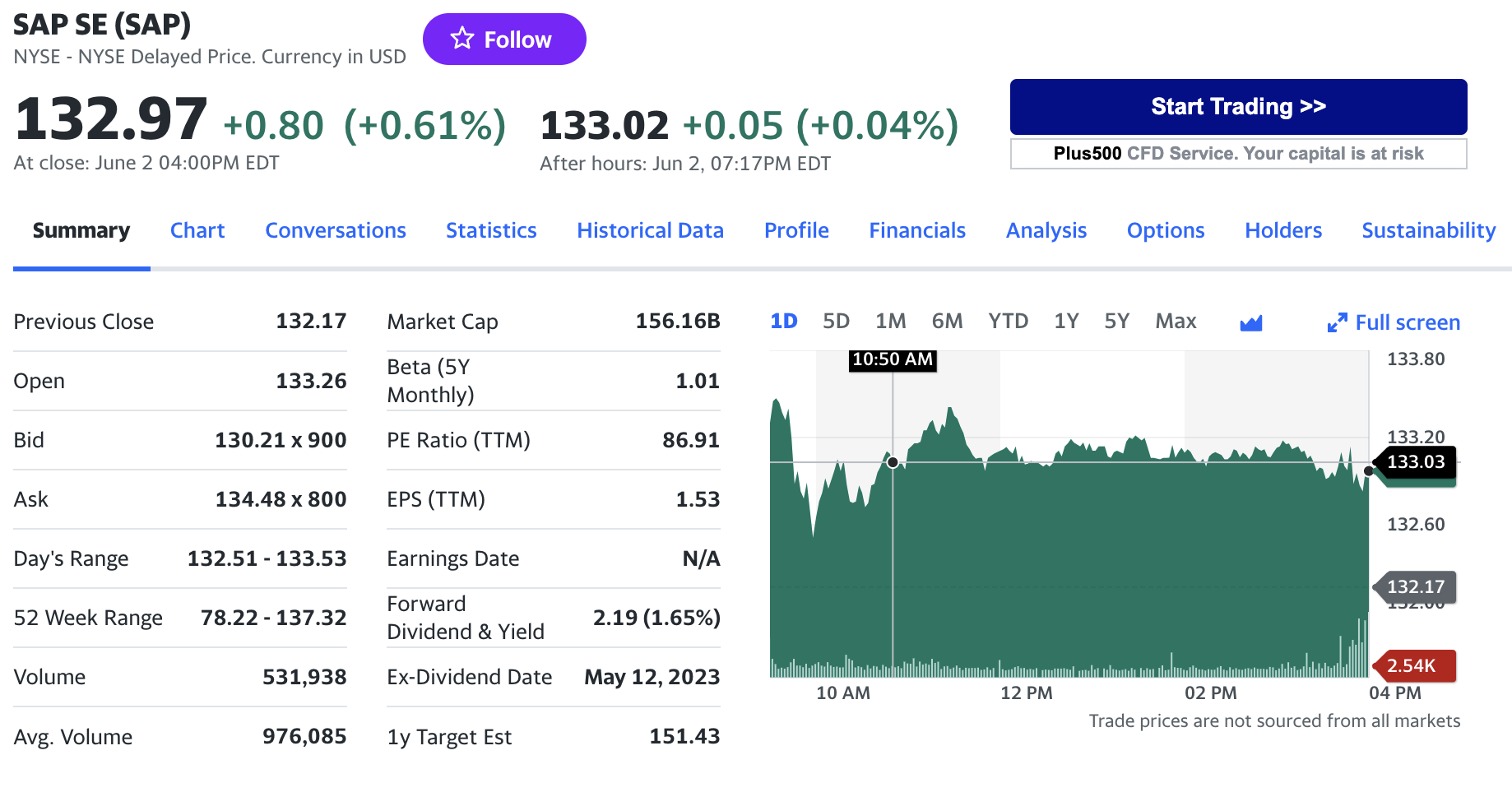This detailed image caption outlines the stock performance and financial data of an unspecified company. The current stock price is 10.003.002, showing an increase of 0.05% with an additional rise of 0.04% in after-hours trading as of 7:17 PM. The stock is part of a popular index ("blue oval"), and recent trading activities include an increase of plus 500 in trading volume. Key points of interest include the company's focus on safety, services, recoverables, and risk management. The interface displays a comprehensive summary encompassing charts, conversations, statistics, historical data, financials, analysis, options, holders, and sustainability metrics.

The previous closing price was 132.7, with an opening price of 133.26. The bid stood at 138.21 by 900 shares, and the days range fell between 132.51 and 133.53. The highest price recorded was 133.52, with a recurring value of 78.22, and the peak volume at 137.32. Key financial metrics include a market cap of 156.6 billion, a beta of 1.01, and a beta ratio of 69.1. The APS is 1.43, with the earnings date still yet to be announced (N.S.A.). The forward dividend yield is 2.19, equating to 1.68%, with the ex-dividend date on May 12, 2023. The one-year target estimate stands at 15.443. The report concludes with a timeline of activities on Monday, the 5th of September, noting continued market involvement from 1 PM to 6 PM.